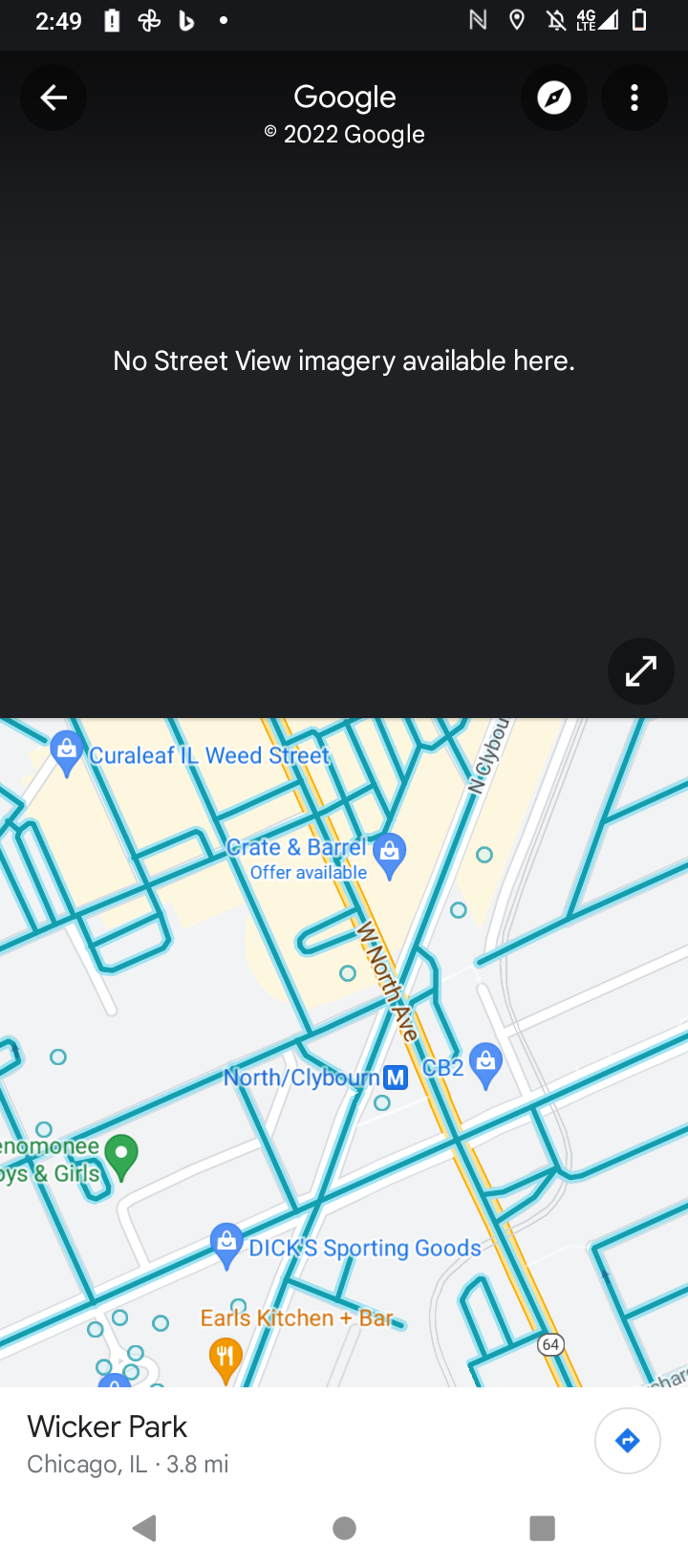Screenshot of a smartphone Google Maps display at 2:49 PM, showing Wicker Park, Chicago, Illinois. Battery level is low. The top of the image shows a black banner with the message "No Street View imagery available here." The map highlights key locations: the North and Clybourn Metro stop, Crate & Barrel (with an offer displayed), Curaleaf Illinois (a cannabis dispensary), Dick's Sporting Goods, and Earl's Kitchen and Bar. Despite the map indicating clear traffic, local knowledge suggests this is unusual for the area.